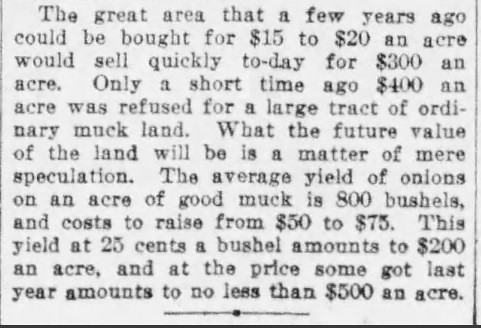The image is a grainy close-up of a printed text excerpt, likely from a newspaper advertisement. The text, in dark black ink against a white-to-gray background, reads: "The great area that a few years ago could be bought for $15 to $20 an acre would sell quickly today for $300 an acre. Only a short time ago, $400 an acre was refused for a large tract of ordinary muck land. What the future value of the land will be is a matter of mere speculation. The average yield of onions on an acre of good muck is 800 bushels and costs to raise from $50 to $75. This year's yield at 25 cents a bushel amounts to $200 an acre, and at the price some got last year, amounts to no less than $500 an acre." At the bottom of the text, there is a short black line with a black dot in the middle, adding to the visual detail of the grainy image.